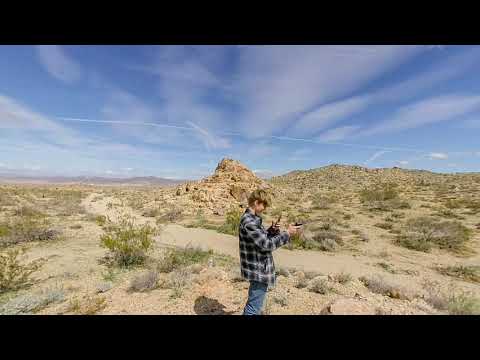In this vibrant outdoor photograph, a young, college-aged person with blonde hair stands alone in a sprawling desert landscape, looking downward at his phone, possibly taking a selfie or FaceTiming. He is dressed in blue jeans and a long-sleeved black and white plaid flannel shirt. The desert environment is expansive, featuring rocky, dry land interspersed with sparse green shrubs and patches of dead grass, creating a predominantly yellowish-brown terrain. A faint dirt path runs through the scene, leading the eye towards the distant horizon where brown mountains rise subtly against a bright blue sky. White streaks of clouds, possibly jet streams, stretch across the sky, adding contrast to the sunny, warm day. The setting evokes a sense of isolation yet serenity, typical of a desolate area that might be found in Arizona.